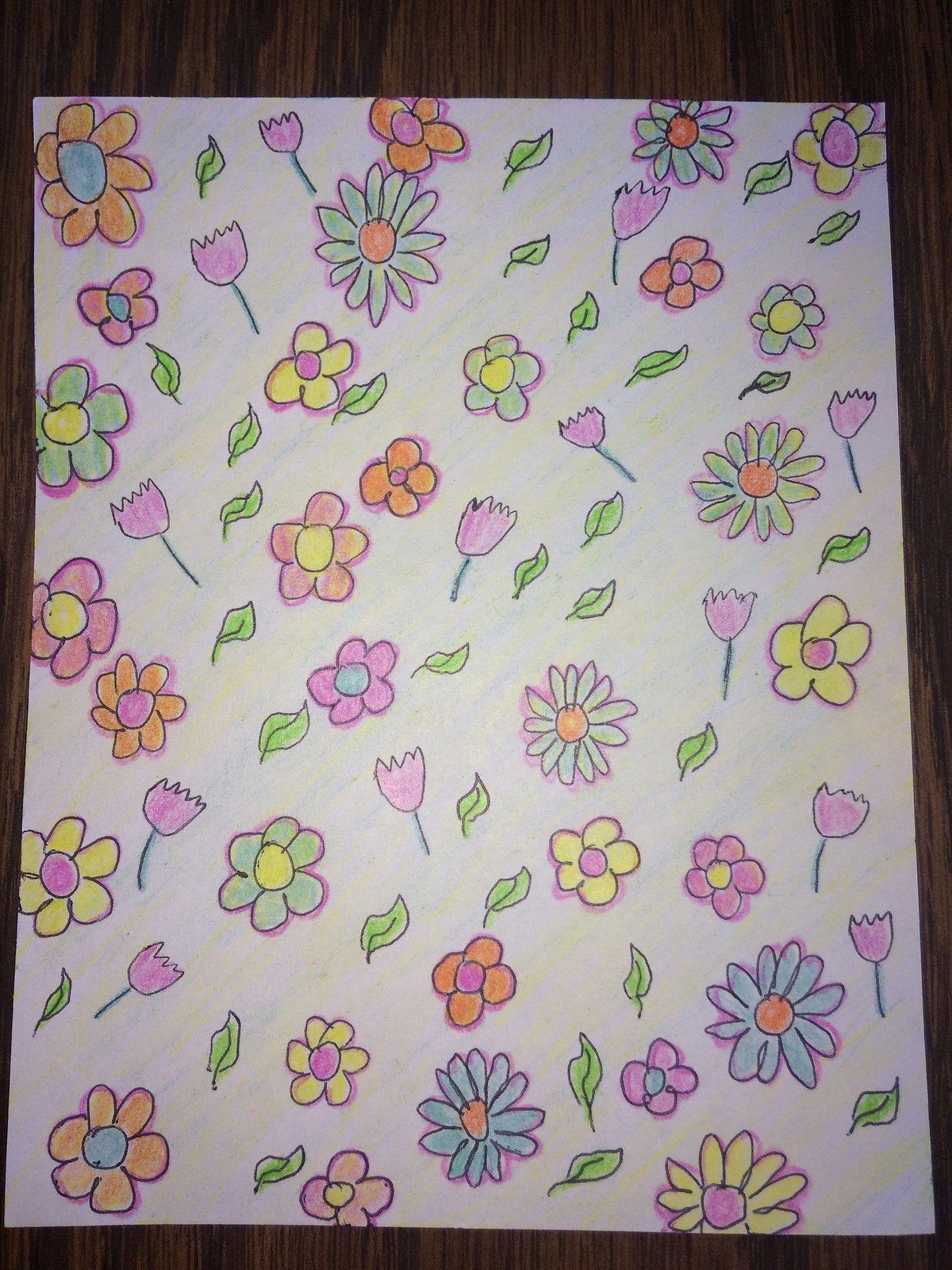This is a detailed photograph showcasing an intricate piece of hand-drawn artwork laid on a dark wooden surface. The image appears to have been captured using a flash, highlighting the fine details of the illustration. The artwork features an array of delicate flowers, each meticulously outlined in pink, with petals rendered in a vibrant palette of colors including orange, green, pink, and yellow. The diversity in floral species is evident, with daisies and tulips among the varieties depicted. Scattered between these blossoms are small, solitary green leaves, adding to the whimsical and natural pattern. The background of the drawing boasts a subtle blend of bluish and yellowish hues, achieved through careful shading, which gives the piece a unique depth and prevents the white paper from appearing stark. The medium used for this creation seems to be colored pencils, given the precision and texture observed. The entire page is densely populated with flowers and leaves, reminiscent of an elaborate, beautifully designed wrapping paper.